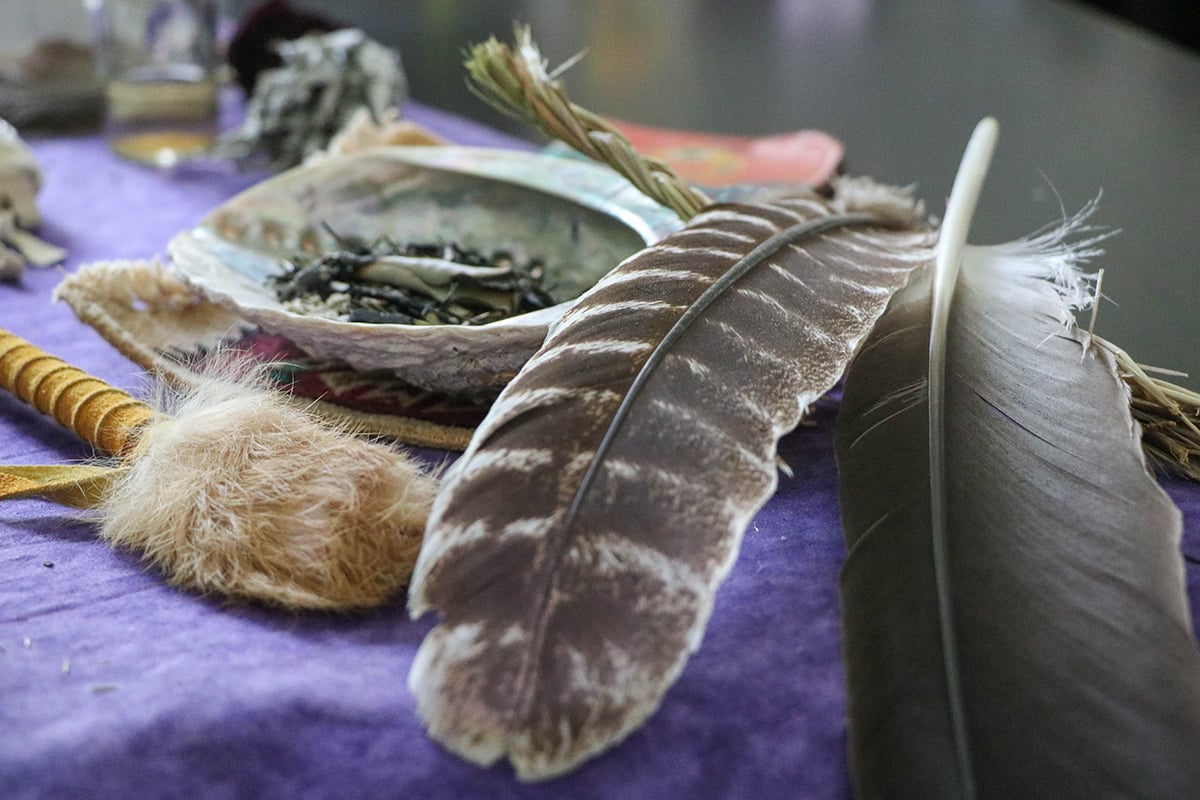This horizontally oriented, realistic photograph features a table draped in a purple cloth, set against a muted gray background. Dominating the scene are various Native American healing tools, meticulously arranged in the center of the image. Two prominent brown feathers with white stripes lay on the right side, alongside another feather with a dark gray underside. A beigeish-gray bowl sits on the table, filled with green herbs, suggesting a connection to natural remedies. To the left, a stick wrapped in leather and adorned with fur — possibly a rabbit's foot — highlights traditional craftsmanship. An additional collection of sacred objects rests within an abalone shell, reinforcing the cultural significance. A glass of water stands in the background, while twine and rope add texture to the setting. The combination of these elements, from woven sticks to possible ceremonial items, implies a display of Native American medicine tools, potentially curated for educational or museum purposes.